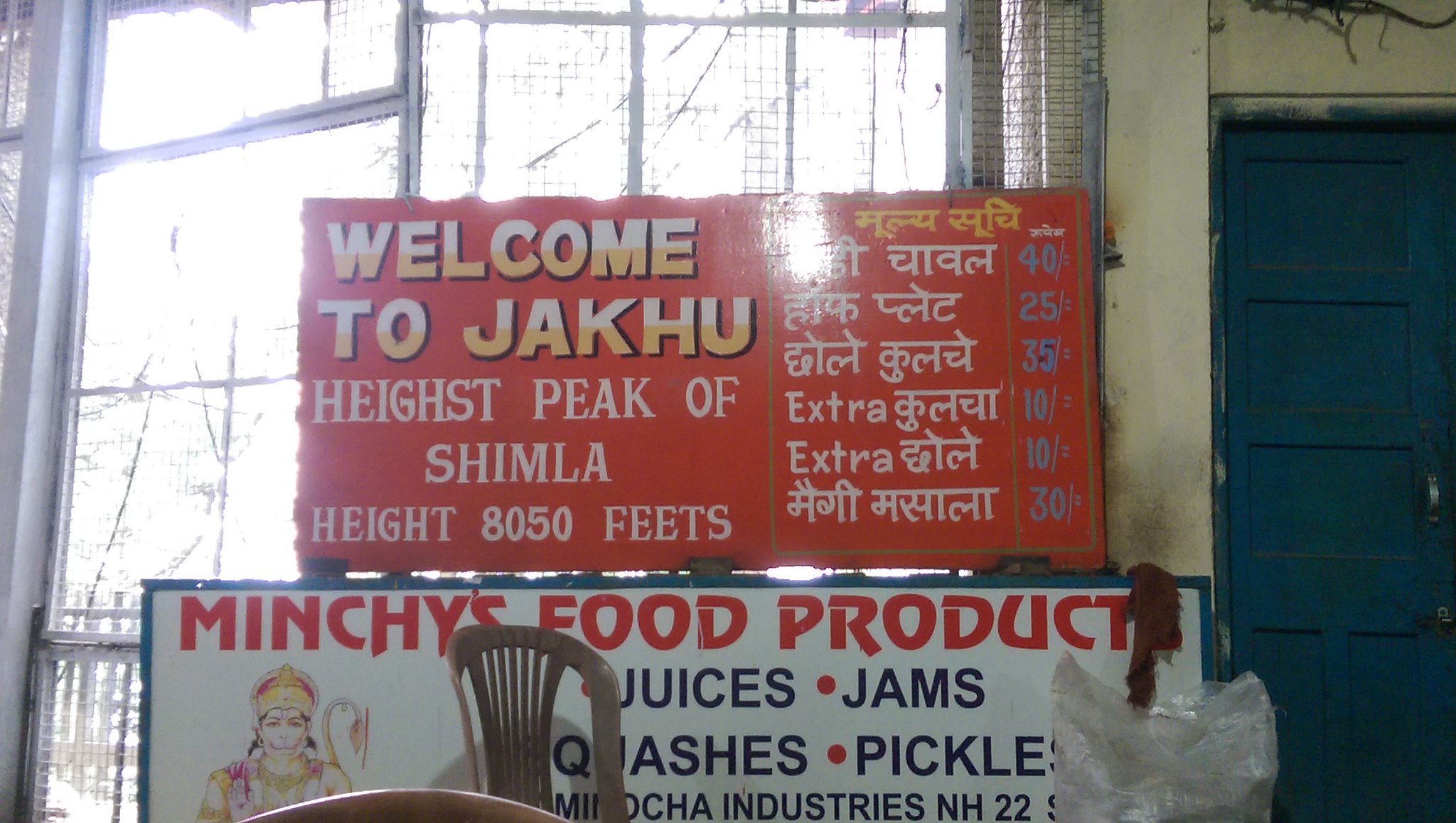The image depicts an indoor setting that appears to be a produce store, brightly illuminated by an overcast daylight filtering through a window in the background. Centrally positioned in the scene are two prominent signs. The top sign is red with white and yellow text reading, "Welcome to Jakku, highest peak of Shimla. Height 8,050 feet." On its right side, there's additional text in an Asian script. Below it is a white rectangular sign with red writing stating, "Minchie's Food Products," followed by the list of items: juices, jams, squashes, pickles, and listing "Minocha Industries NH-22." This sign also features a picture of Hanuman with gold attire on the left side. A brown plastic chair is placed in front of the signs. To the right of this display is a blue wooden door, contrasting with the dirty white wall adjacent to it. The colors in the image span a spectrum, including blue, tan, black, red, purple, yellow, orange, light blue, white, and gray, giving the scene a vivid and somewhat eclectic appearance.